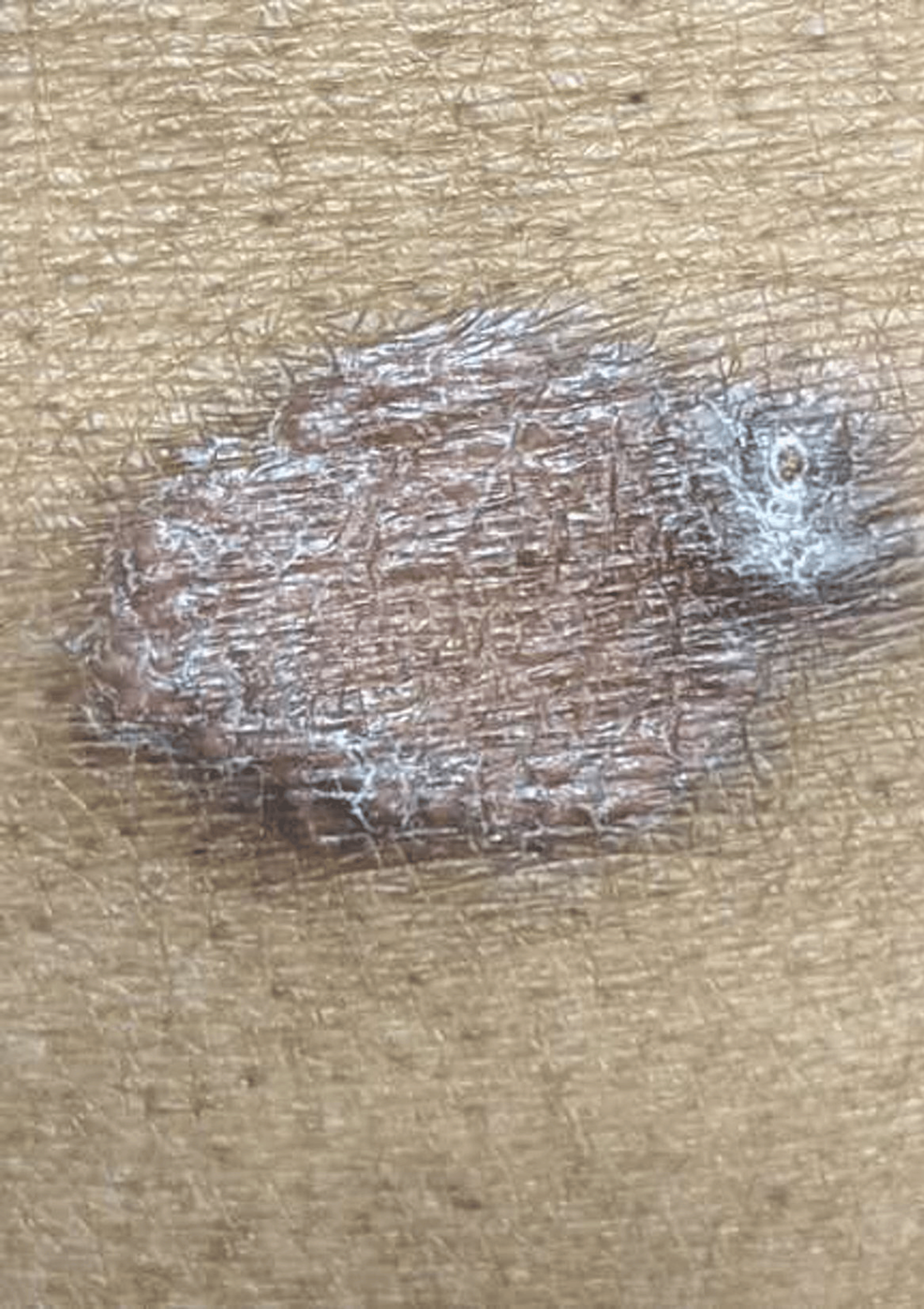This close-up image reveals a detailed view of a possibly unhealthy mole on Caucasian skin. The mole, positioned in the center, appears circular with distinctive grayish and light skin pinkish tones. On its right edge, there is a prominent white blob that stands out, slightly elevated above the surface. The surrounding skin is characterized by deep, pronounced wrinkles and numerous brown freckles, giving it a yellowish hue interspersed with brown lines and dots. The mole itself exhibits brushed gray areas extending towards the right edge of the picture, while the left side has a rounded contour. The overall appearance of the mole is slightly raised and irregular, suggesting an unhealthy nature. The background displays a texture that some might liken to neural patterns, adding to the complexity of the image.